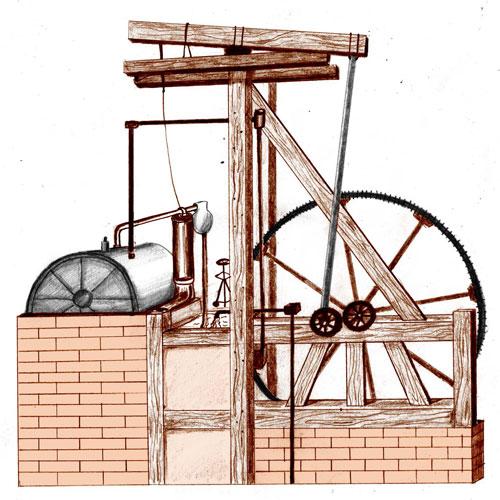The image features a detailed illustration of an antique contraption set against a white background, with no visible border. At the base of the apparatus, there is a partial brick wall from which wooden poles and planks extend, forming a supportive framework that crisscrosses and stabilizes the structure. On the right side, a large, jagged metal wheel, possibly a gear, is prominent. Beside it, there are several smaller gears indicating a complex mechanical function. To the left, a metal container rests on top of the framework, connected by strings and wooden components, adding to the intricate design. The setup also includes some copper piping leading into what appears to be a metal still, suggesting a use for liquid processing. Together, these elements hint at a piece of primitive machinery, perhaps reminiscent of an old-fashioned ironing mangle or a rudimentary moonshine still or smoker. A stool in the background implies manual operation, where the user might press down on a plunger to activate the mechanism, setting the gears and rolling cylinder into motion. The intricate depiction, though complex, underscores the antiquated and industrial essence of the device.